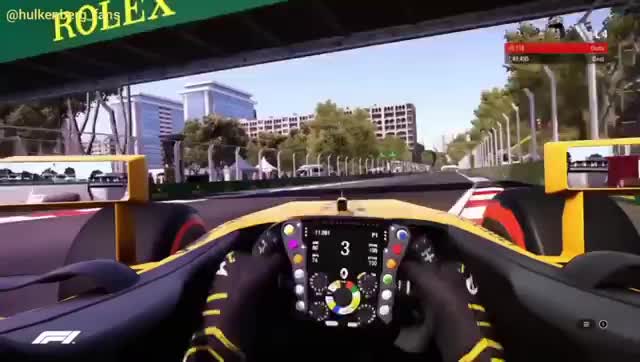The image appears to be a detailed snapshot from a racing video game. In the top left corner, there's a green banner with the word "Rolex" prominently displayed in yellow. The scene features the underside of a bridge, contributing to the immersive experience of a race track environment. The perspective suggests that the viewer is inside a race car; the bottom of the image shows a steering wheel framed by hands wearing black gloves with yellow accents. A digital indicator displays the number "3" on the screen in front of the driver. The roadway stretches ahead, bordered by fences on both the left and right sides, with rows of trees beyond the fences. The blue sky provides a serene backdrop, contrasted by two silver rectangular buildings in the upper left and a white rectangular building slightly to their right. At the top right of the image, there are red and black banners, though their text is indiscernible.